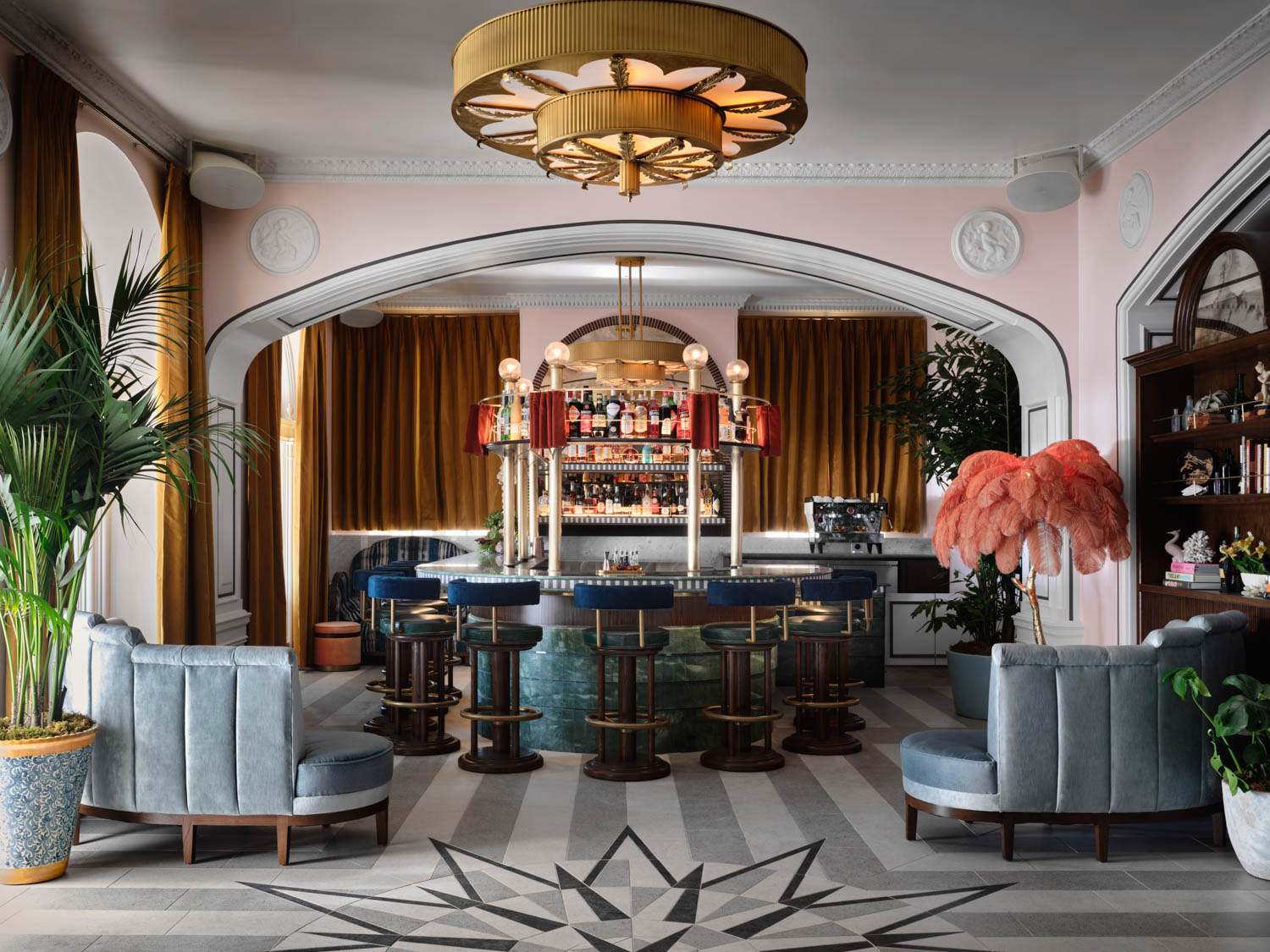This detailed image captures an indoor Art Deco-inspired bar and lounge area, set in what appears to be a luxurious room within a house. The primary focus is a centrally positioned, horseshoe-shaped bar adorned with a distinctive blue-green stone bottom and dark wood accents, topped with a striking blue and white striped counter. Surrounding this elegant bar are several barstools with dark blue leather backrests and darker green leather cushions, complemented by brass bars and dark wooden legs.

The bar features an elaborate three-layered shelving unit at the back, stocked with various liquors, and additional liquor bottles creatively displayed above the bar, emphasizing the array with labels facing outward. The bar area is illuminated by tall columns with lights on top and a prominent brass chandelier resembling a wagon wheel, adding to the sophisticated ambiance. 

The room's flooring showcases an intricate, geometric, star-patterned carpet in shades of gray, off-white, and tan. The walls are softly painted pink, adorned with sconces in the corners, and there are large gold curtains framing the bar area. An espresso machine is situated on a bench to the right of the bar, and luxurious gray couches with an inward arch are arranged on either side of the space, further accentuating the inviting and well-designed lounge atmosphere.